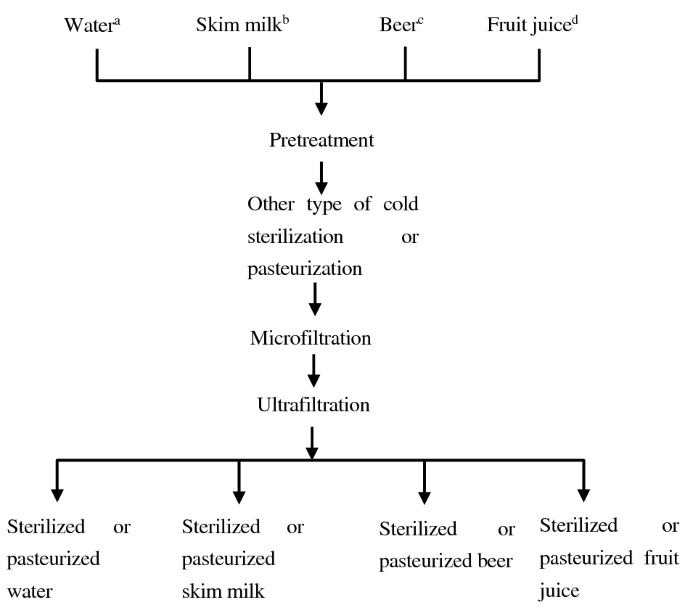The black and white illustration depicts a detailed flowchart of the filtration and sterilization process for four different beverages: water (A), skim milk (B), beer (C), and fruit juice (D), each indicated by corresponding letters. These inputs converge into a single down arrow labeled "pre-treatment," followed by a sequence of processes: "other type of cold sterilization or pasteurization," "microfiltration," and "ultrafiltration." After undergoing these steps, the flowchart branches out into four distinct outputs: sterilized or pasteurized water, skim milk, beer, and fruit juice. The image appears to be a textbook-style breakdown of the different filtration methods utilized to prepare these beverages.